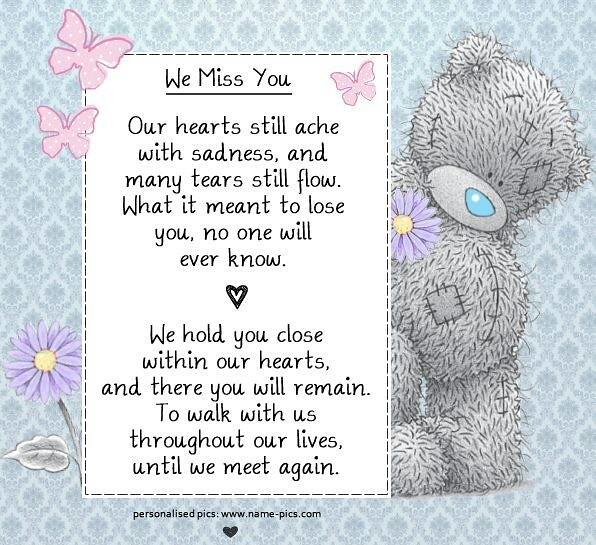This square image, reminiscent of a sympathy card, features a poignant and heartwarming design. The backdrop is a blue and gray diamond pattern that gives a soft and comforting visual appeal. A light gray teddy bear with a blue nose, adorned with stitches and patches, sits on the left side looking melancholic. Interspersed within the background are two purple flowers, each with vibrant yellow centers, enhancing the tender theme.

Central to the image is a white rectangle bordered by a dotted line, containing a heartfelt poem. The poem begins with the words "We miss you" in bold, underlined black letters, and continues with, "Our hearts still ache with sadness and many tears still flow. What it meant to lose you no one will ever know. We hold you close within our hearts and there you will remain to walk with us throughout our lives until we meet again." A small heart symbol follows this touching message.

Adorning the top edges of the white rectangle are three pink butterflies, with an additional butterfly on the top right-hand corner of the card, symbolizing transformation and hope. Below the rectangle, against the blue patterned background, is the source of this beautifully crafted message, inscribed as "Powerful Pics" along with a website name in small black letters, accompanied by a black heart symbol. This card is a delicate and moving tribute to the memory of a loved one, suitable for sharing in both print and digital formats.